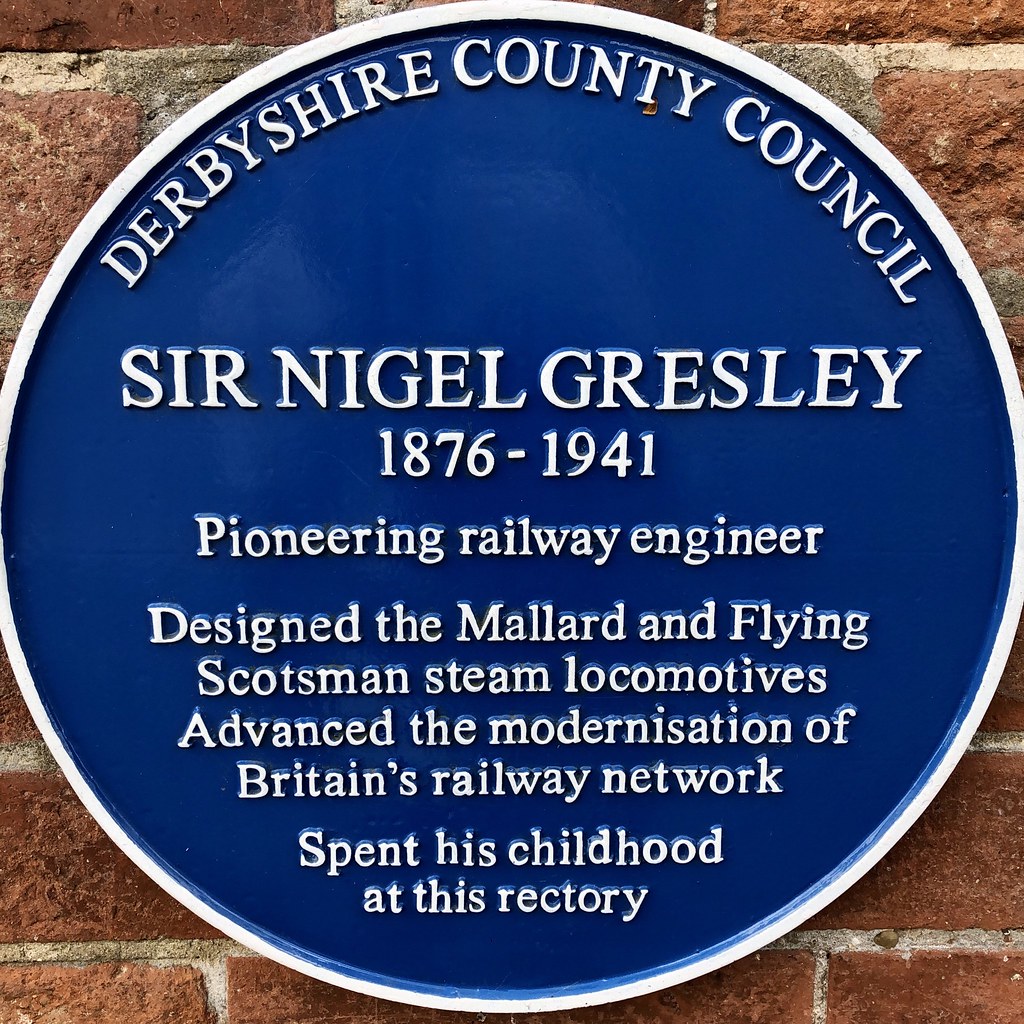The photograph depicts an outdoor iron marker, approximately six inches square, mounted on a red brick wall with light-colored grout. At its center is a large, round blue metal plaque framed by a raised white border. The sign features white text that reads: "Derbyshire County Council" in a semi-circular fashion from the 10 o'clock to the 2 o'clock positions at the top. Beneath this, it prominently states "Sir Nigel Gresley, 1876 to 1941" in all capital letters. The plaque pays homage to Sir Nigel Gresley, a pioneering railway engineer who designed the iconic Mallard and Flying Scotsman steam locomotives and advanced the modernization of Britain's railway network. It also notes that Gresley spent his childhood at the rectory where the marker is placed, serving as a memorial to his contributions. The detailed blue and white sign stands out against the red brick background, making it a notable outdoor memorial.